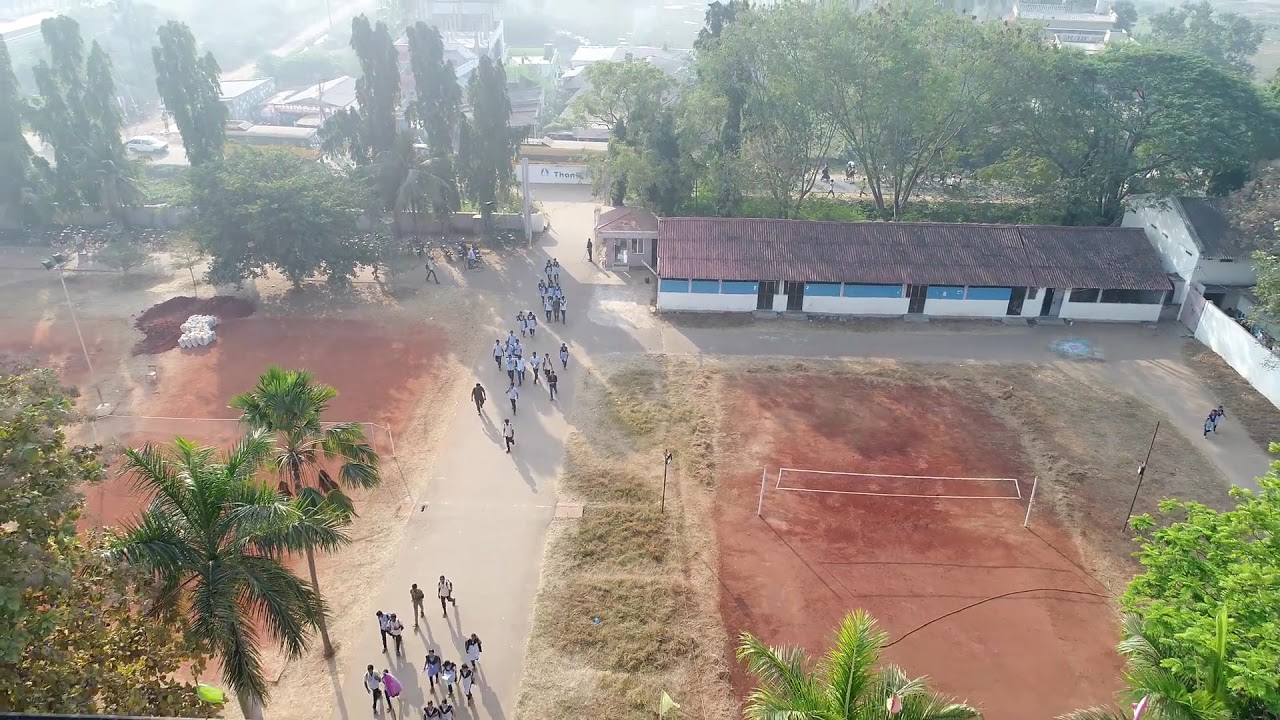This overhead photograph captures a vibrant scene on what appears to be a school campus or a campground in a tropical or subtropical region. A gray pathway extends from the bottom edge of the image towards the top, populated by numerous people, possibly students in white uniforms, walking along it. Flanking this pathway, on the right side of the image, is a red clay volleyball court complete with a net, in front of a low, white-and-blue building with a dark roof that could serve as locker rooms, bathrooms, or a small lodge.

To the left of the pathway, there might be another red clay court, perhaps for tennis or volleyball. The scene is dotted with green foliage, including several palm trees in the bottom corners of the photograph. In the background, there is a densely wooded area leading up to what seems to be the outskirts of a town, visible through the tops of various buildings and houses. The overall scene is bustling with activity, framed by a mixture of natural and built environments.